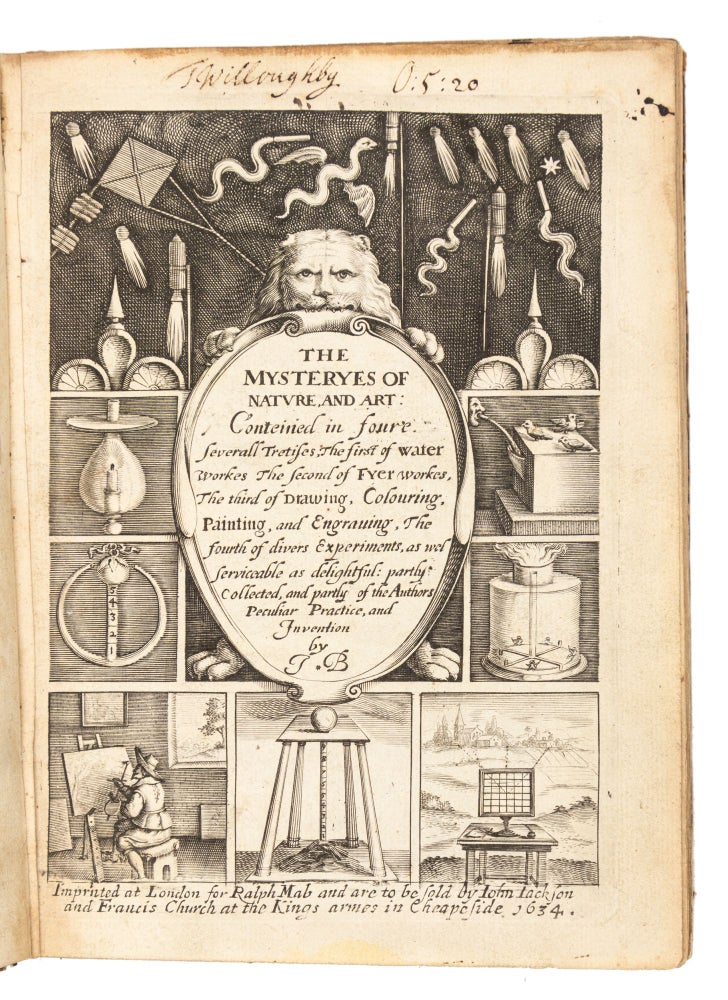The image appears to be an old, yellowed page from a book, possibly dating back centuries. At the very top, there is a handwritten inscription in black cursive that reads "T. Willoughby 0520." The central focus of the page is a detailed, black-and-white illustration featuring a lion's head with its paws placed on an oval, mirror-like object. Inside this object is text in Old English spelling that reads "The Mysteries of Nature and Art contained in four several trifles, the first of water works." Surrounding this central image are a series of smaller illustrations arranged like comic book panels. These depict various items and contraptions, including art devices like brushes and pointed tools, a clear encasement, a person painting at an easel, and other ambiguous objects. One notable image includes what appears to be a screen monitor with an old town city and a church steeple in the background. At the bottom of the page is a paragraph in hard-to-read script, indicating the publication details: "Imprinted at London for Ralph Mab, and to be sold by Francis Church at the King’s Arm in Cheapfide 1634."